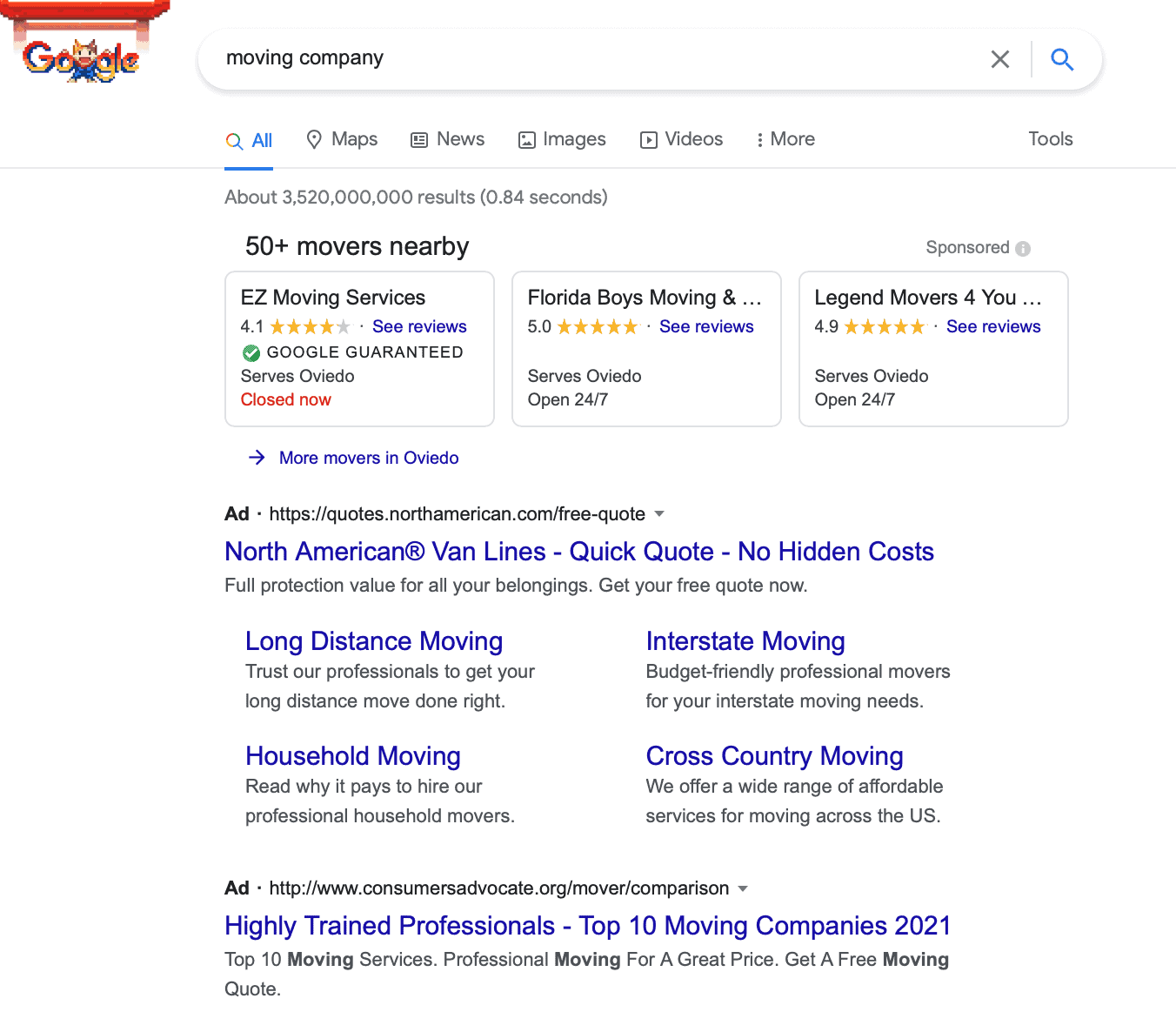The image depicts a Google search results page featuring a custom Google logo at the top. This special logo consists of an orange bar at the top, with two bars extending downward and another orange bar crossing horizontally beneath them. In the center of the logo is a small cartoon character. 

The search query entered in the search box on the left side of the screen reads "Moving Company." To the right of the search box, there is an 'X' button, a vertical line, and a blue magnifying glass icon for initiating the search. Below this section, there is a multi-colored magnifying glass icon with tabs for different search categories such as "All," "Maps," "News," "Images," and "Videos." The "All" tab is active, indicated by a blue line beneath it. There's also a "More" option indicated by three dots, and a "Tools" button located on the far right.

The search results indicate approximately 3,520,000,000 results, found in a swift 0.84 seconds. The page highlights "50+ movers nearby," presenting three companies in boxed sections: Easy Movers Service, Florida Boys Moving, and Legend Movers For You. Each company listing includes star ratings. The first has a green circle with a checkmark labeled "Google Guarantee." It notes the operational status of each mover: "Closed Now" in red for the first, while the second and third state "Open 24-7."

Below these featured movers is the option "More Movers." There's also a listing for "North American Van Lines®" with a tagline, "Quick Quotes, No Hidden Costs," followed by various service categories highlighted in blue such as "Long Distance Moving," "Household Moving," "Interstate Moving," and "Cross Country Moving," each accompanied by brief, black text descriptions.

Additionally, there's an advertisement for a website titled "Highly Trained Professionals - Top 10 Moving Companies 2021," with further descriptive text in black beneath it.